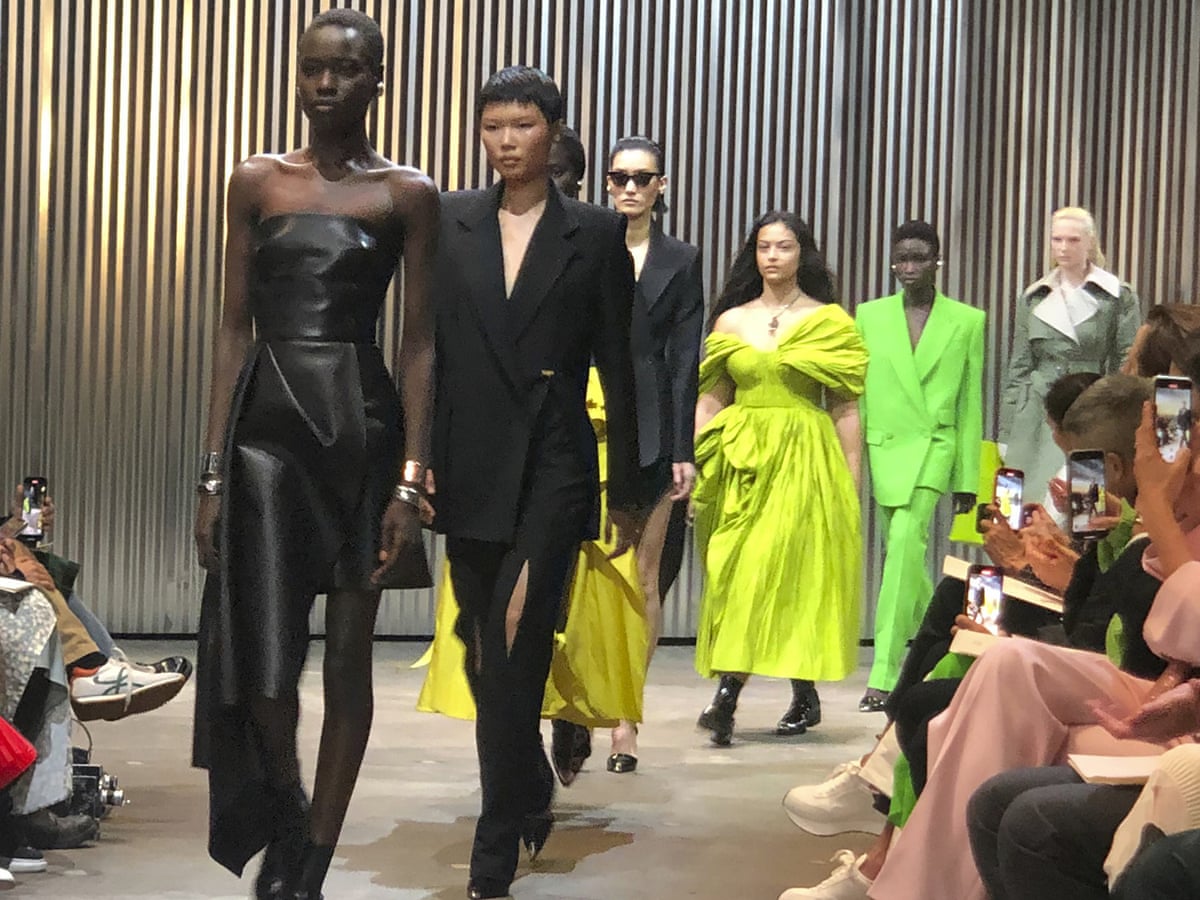The image captures the vibrant scene of a fashion runway show. Models gracefully stride down the catwalk, flanked by the attentive audience whose knees are visible along the edges. At the forefront, a tall and elegant Black woman commands attention in a sleek black catsuit, accentuated by silver bangles on her wrists. Beside her, an Asian woman exudes sophistication in a black trouser suit featuring a side split above the knee.

Further back, a figure is barely discernible in a bright yellow ensemble, their details obscured. Just behind, another model showcases a grey suit with a split skirt, maintaining the show’s chic aesthetic. Following her, a striking off-the-shoulder acid yellow dress is worn by a woman with long, flowing black hair, capturing eyes as it moves.

The progression continues with a model donning a pale green suit, another elegant ensemble worn by a Black woman. Bringing up the rear, a second white model presents a fashion-forward grey raincoat with contrasting beige lapels. The backdrop of the scene is set against a stripy grey curtain, adding a sophisticated touch to the overall atmosphere.